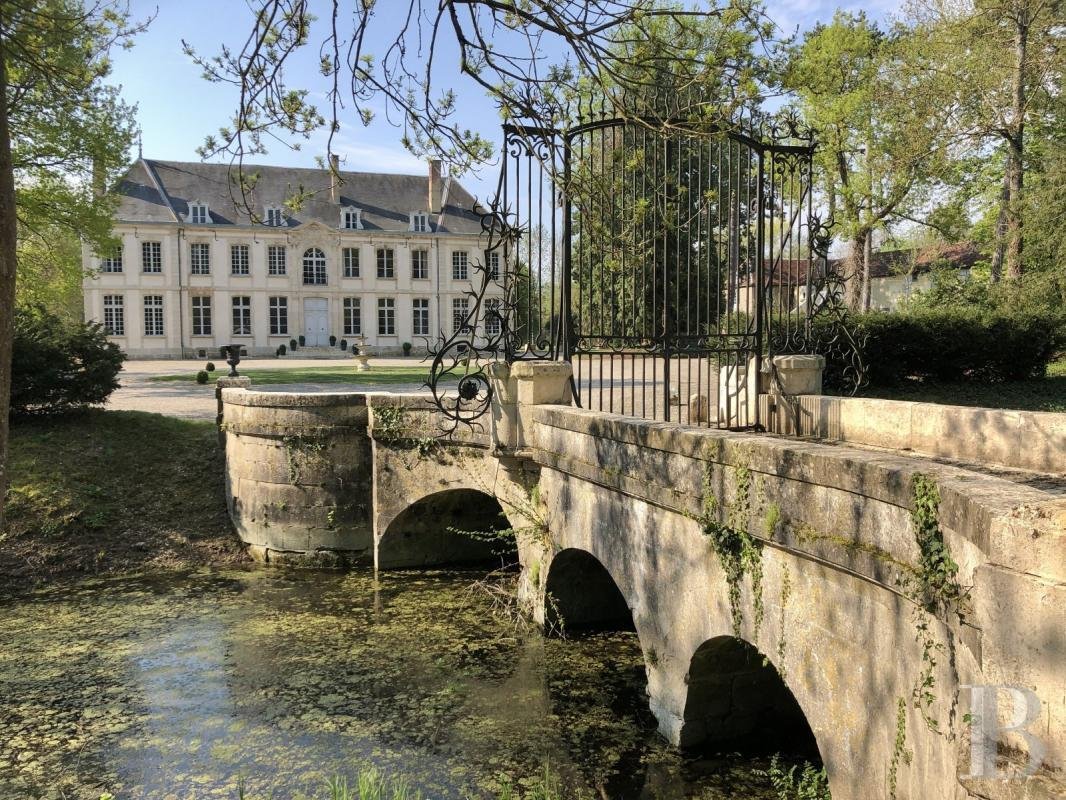The image showcases a grand, old white mansion with a long, rectangular facade. The mansion features a greyish roof adorned with a few chimney stacks—one clearly visible on the top right and possibly another obscured by trees on the left. The structure boasts numerous windows, approximately 10-11 on each floor, and a central white door at the bottom. 

In the foreground, a small courtyard with a circular patch of green grass, possibly containing a fountain, leads to a driveway or walkway. This path extends outward to a prominent stone bridge, which occupies the right-hand side of the image and serves as the focal point. The bridge, constructed with old stone bricks, features three arch supports and spans a small, murky creek or river.

A tall, imposing metal gate, designed to prevent unauthorized access, blocks the entrance to the mansion from the bridge. Surrounding the scene are green, budding trees that indicate springtime and frame the mansion against a bright blue sky, suggesting the photograph was taken on a clear, sunny day. The image captures the blend of the mansion's stately presence with the serene natural elements around it.